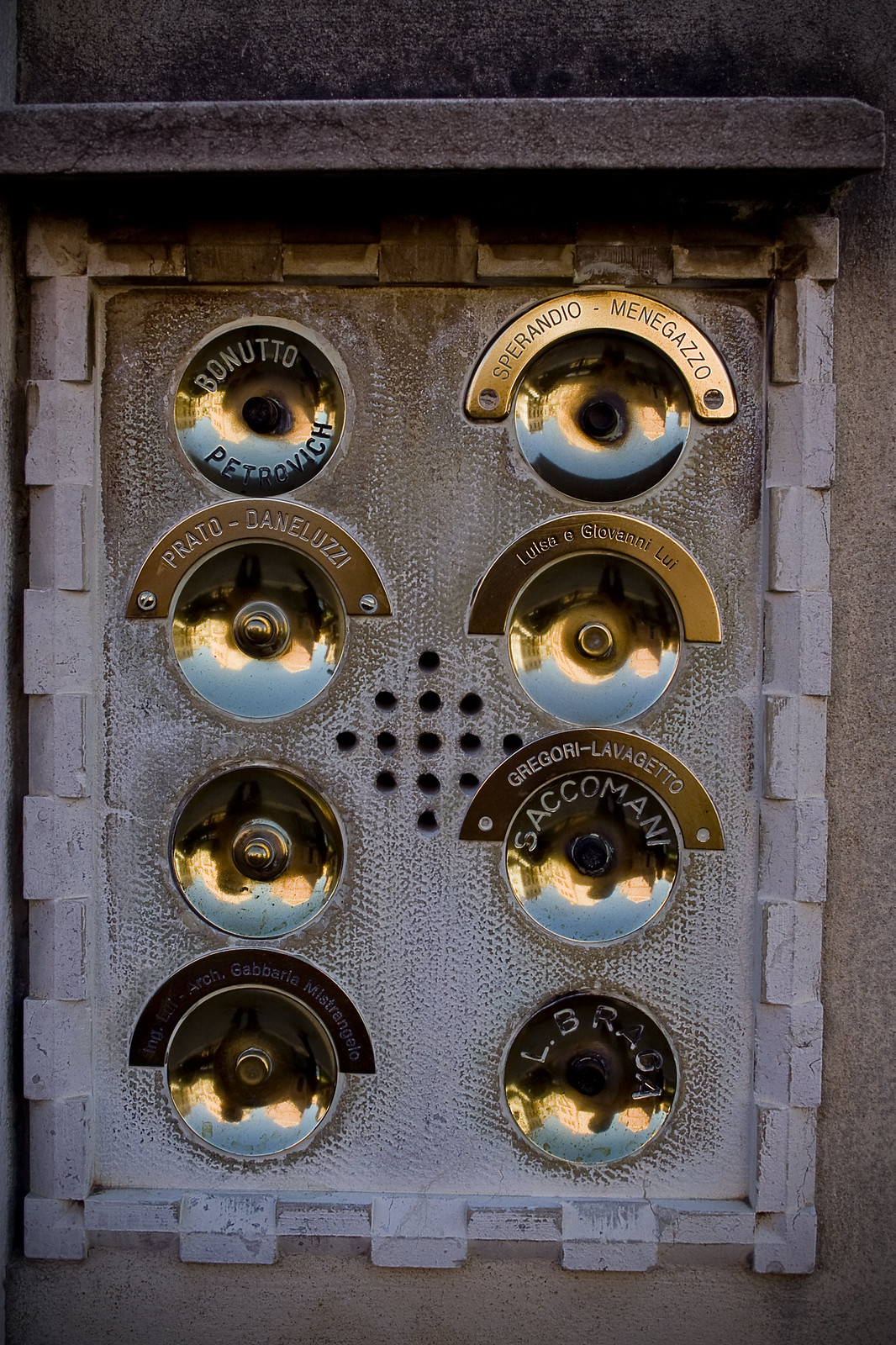The photo depicts a well-weathered call box or intercom system seamlessly integrated into a smooth tan stone wall. The centerpiece features an array of functionality and aesthetics: two columns of brass-colored, reflective calling buttons—four on each side—craftily organized around a central speaker grille with 13 small holes. The buttons, adorned with names inscribed in a likely Italian script on half-circle frames, serve as an entry notification system for an apartment building. Each button varies in color, some gold and others black, standing out against the white and brown painted concrete background. Surrounding the white stone frame, which is irregularly segmented, is a darker tan stone that is notably smooth, capped with a dark grey ledge and black stone wall above. A prominent engraved name, "Berondio Menegazzo," can be seen on one of the top placards. The overall condition shows signs of rusting at the top, contrasting with the cleaner whiter sections below, reflecting years of use and exposure.